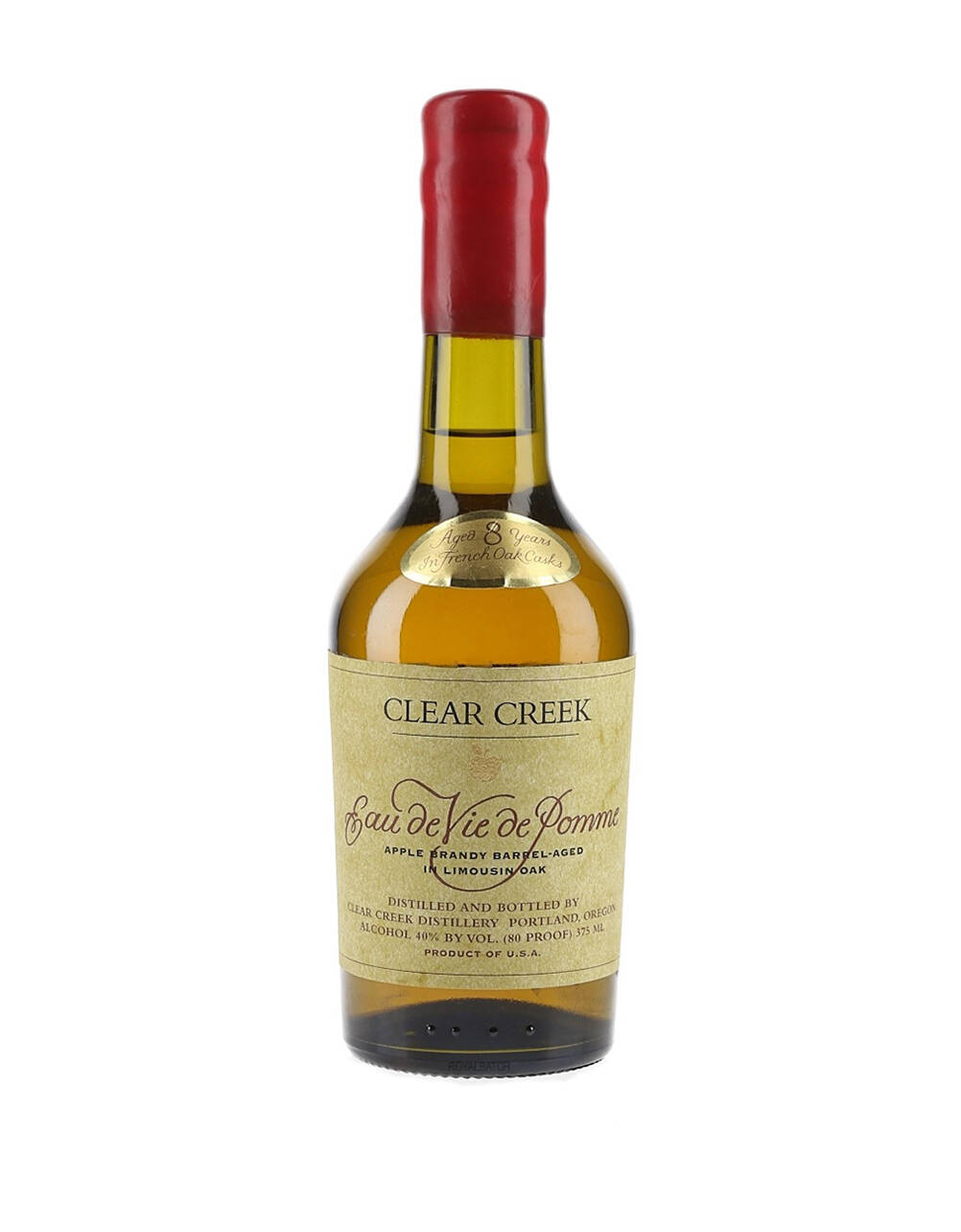The image features a tall, 375-milliliter bottle of Clear Creek Distillery's apple brandy, positioned against a plain white background. The clear bottle has a light yellowish-green tint and contains a golden-colored liquid, reflecting the brandy inside. The bottle's neck is sealed with red wax, extending halfway down, topped by a small, shiny gold sticker indicating it has been aged for 8 years in French Oak casks. The main off-white label reads "Clear Creek" in prominent letters, followed by "Eau de Vie de Pomme" in cursive purple French. Below, it states "Apple Brandy Barrel Aged in Limousin Oak" in English. Further down, the label provides additional details: "Distilled and bottled by Clear Creek Distillery, Portland, Oregon. Alcohol 40% by volume, 80 proof, Product of the USA."